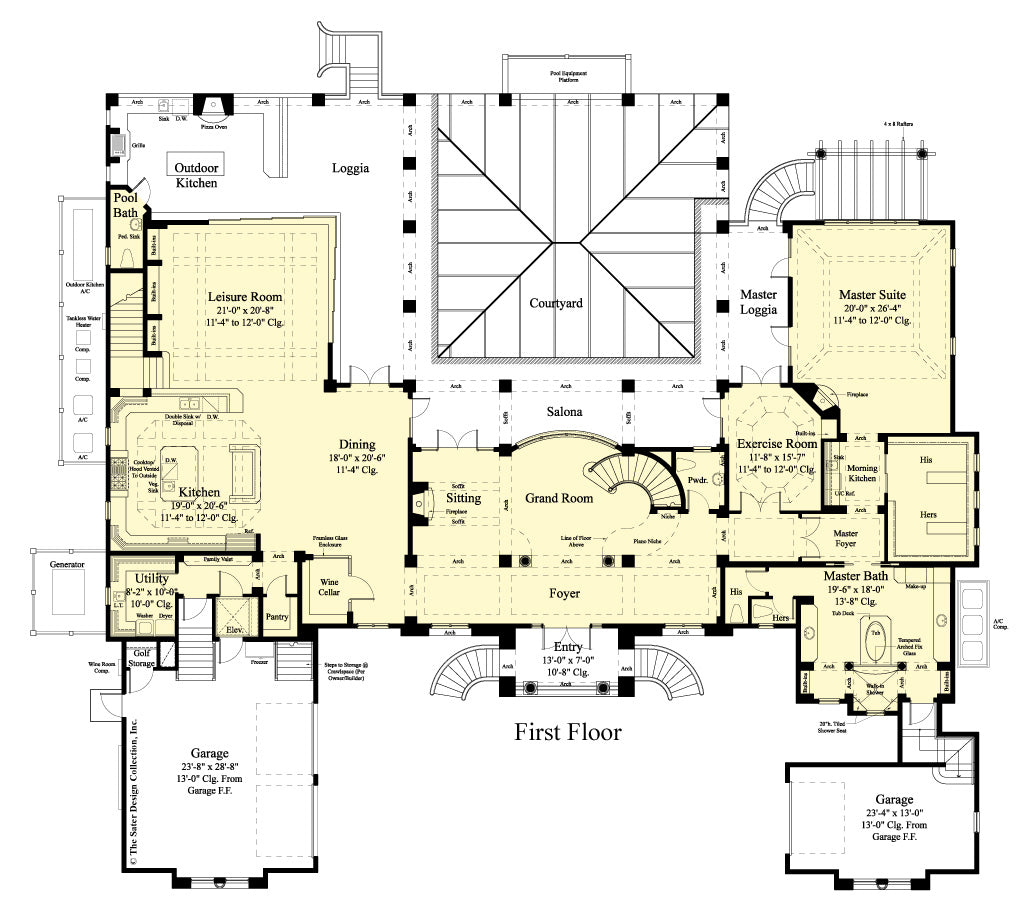This detailed blueprint showcases the first floor layout of an expansive, likely multimillion-dollar mansion. At the bottom of the plan, the entryway leads into a grand foyer, which seamlessly connects to the grand room situated in the middle. Directly above this central space is a square-shaped courtyard, adding a touch of elegance and open-air luxury to the arrangement. On the top right corner, the master suite occupies a prominent position, just above the exercise room, which in turn is located above the master bath. Below the master bath lies one of the garages.

To the top left, an outdoor kitchen stands adjacent to a laundry area positioned to its right, indicating a practical layout. Below the laundry room is the leisure room, providing a relaxing retreat. The kitchen and dining room lie below, with the kitchen on the left and the dining room on the right, designed for ease of access. At the very bottom right of the layout, another garage ensures ample parking space for the residents.

This floor plan reflects an intricately designed and spacious mansion, featuring several specialized rooms including a grand room, leisure room, master suite with accompanying facilities, an outdoor kitchen, and extensive courtyards, making it truly a luxurious residence.